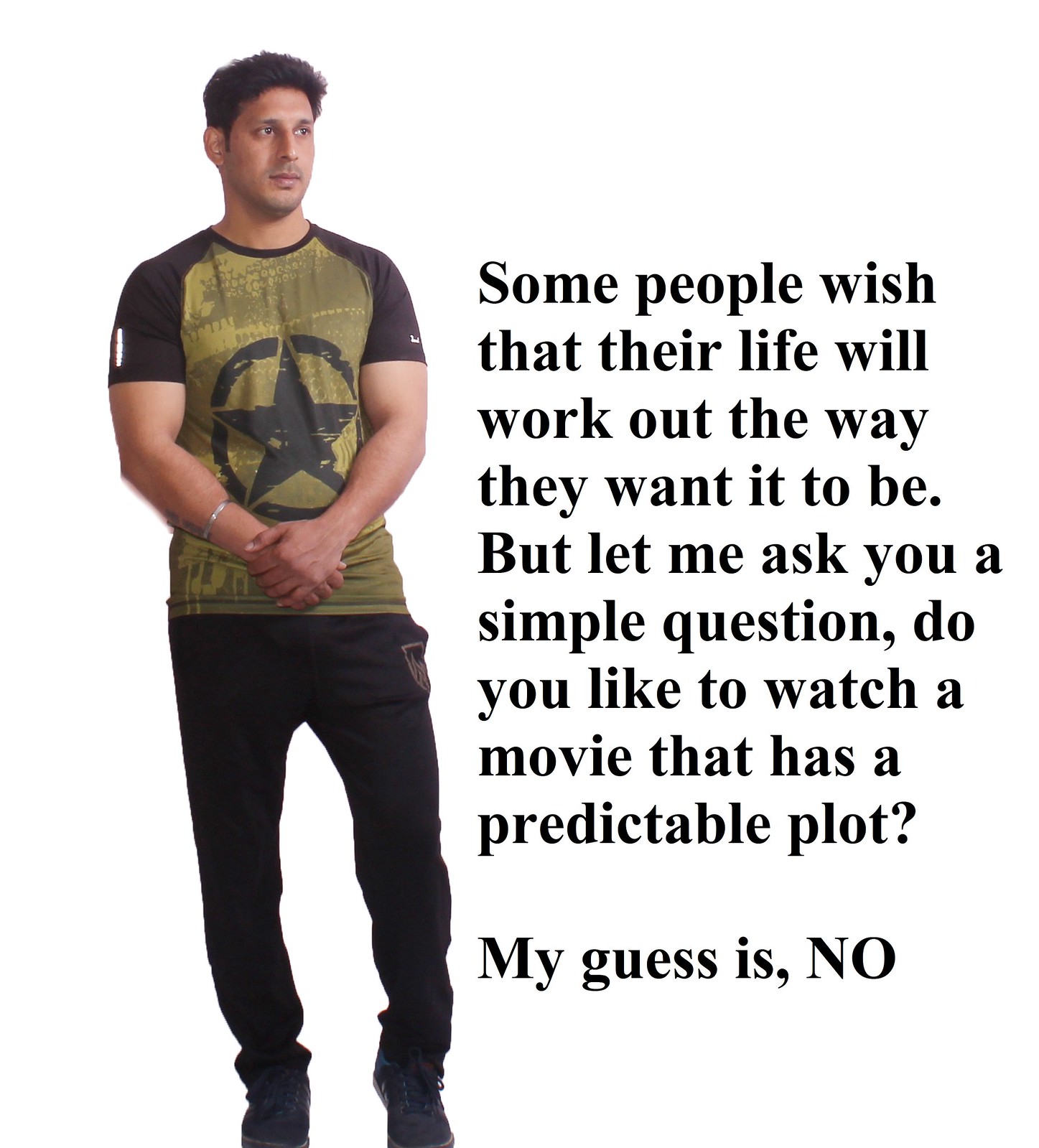In an image set against a stark white background, a man stands to the left of a block of textual content. The man is dressed in a short-sleeved t-shirt with black sleeves adorned with small white symbols. The torso of the shirt is green, featuring a central black star encased in a black circle. He pairs this with black pants and black sneakers. The man has short brown hair, a light facial hair shadow, and a silver bracelet on his left wrist, beneath which a tattoo peeks out. His hands are crossed in front of him, with his left hand resting on top of his right. He gazes thoughtfully into the distance to his right. The text beside him reads: "Some people wish that their life will work out the way they want it to be. But let me ask you a simple question. Do you like to watch a movie that has a predictable plot? My guess is NO," with 'NO' emphatically capitalized. The entire scene, from the man to the text, is superimposed upon the blank, white background, creating a focused and contrasting visual.